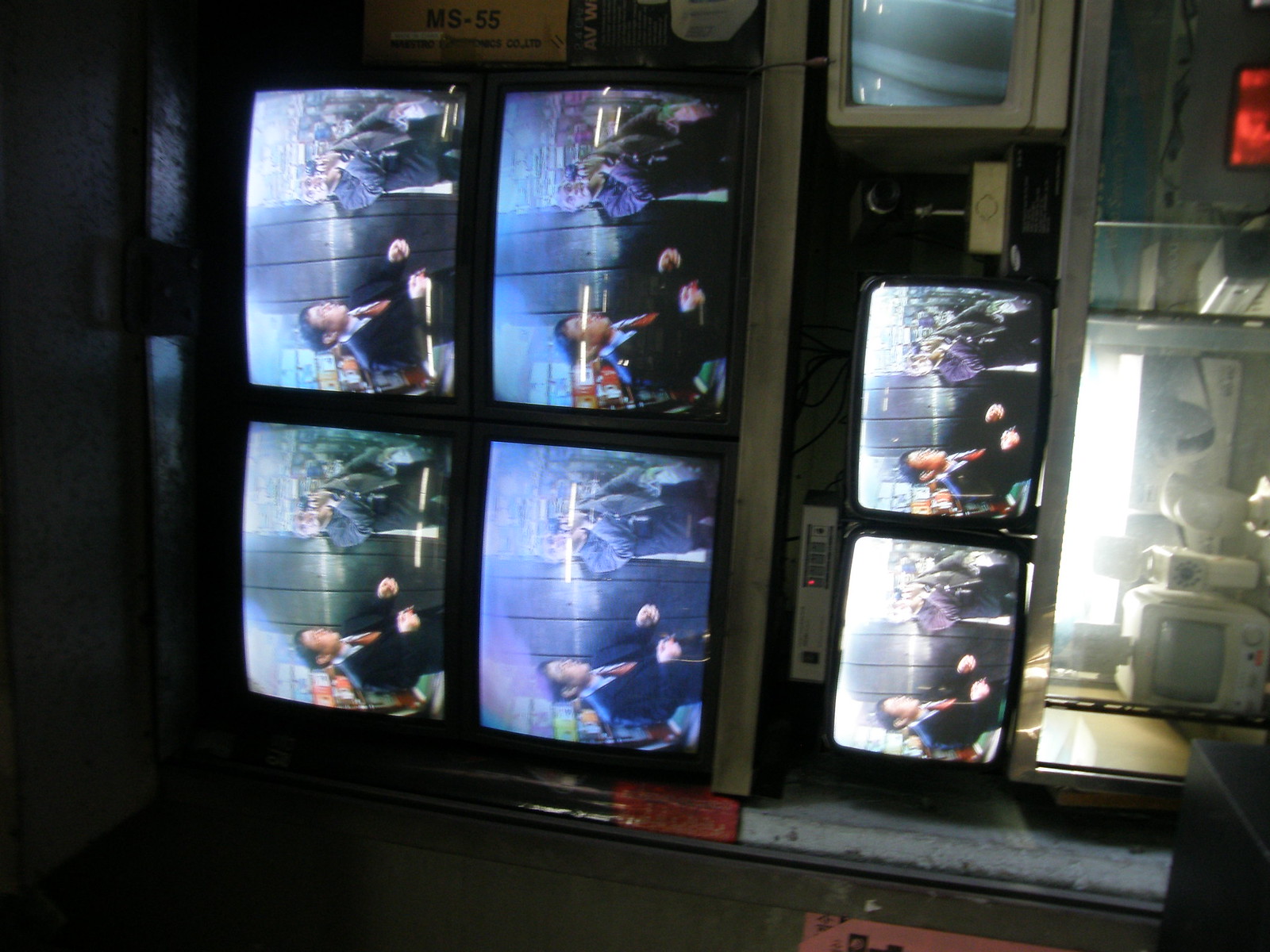The image depicts a chaotic arrangement of vintage tube TVs, stacked one above the other on a metal gray utility shelf that's oriented sideways. There are a total of eight TVs, with the primary set of four being larger and centrally positioned. Each of these larger TVs displays the same somewhat blurry scene: a man in a suit on the left, seemingly interacting with another person in a coat on the right. The screens lack vibrant hues and clarity, indicative of their age. Beneath this main set, two smaller TVs are placed, with one electronic device perched atop them. Among the clutter on the shelf is a tiny white TV, which is turned off, and to its right, an additional monitor with a white frame of unclear function. Surrounding these electronics are various other gadgets, some showing a red light. The background consists of dingy concrete or metal walls painted green and white, reinforcing the utilitarian and vintage atmosphere of the scene.